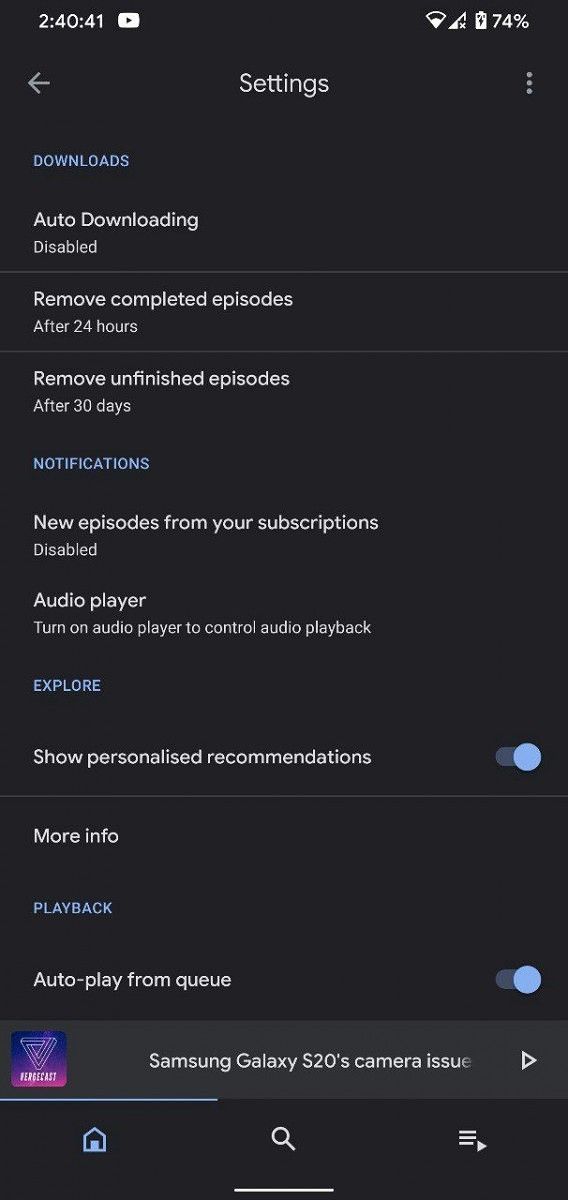This image is a screenshot from a smartphone, featuring various interface elements against a dark gray background. In the upper left corner, white text displays the time as 2:41. Adjacent to this, a white square with rounded corners contains a black triangle pointing right, possibly indicating a video-related app logo, such as YouTube or a similar service.

In the upper right corner, icons denote the phone's status: the battery is at 74% charge, and both Wi-Fi and wireless connection symbols are visible. Central to the top of the screen is the title "Settings" in white font, with a left-pointing arrow symbol of the same color on the left side.

Below, in blue font, the word "Downloads" stands out, followed by white text stating "Auto downloading disabled." Additional information includes settings for removing completed episodes after 24 hours and unfinished episodes after 30 days.

Further down, blue capital letters spell out "NOTIFICATIONS," with text underneath explaining the status of notifications: "New episodes from your subscriptions" is disabled, and an option to "Turn on audio player to control audio playback" is mentioned.

The section titled "Explore" in blue font follows, with an option to "Show personalized recommendations," accompanied by a blue, circular slide button to its right. Below this, "More info" is indicated.

The final category depicted is "Playback," highlighted in blue, featuring the "Auto playback from Queue" option with another blue circular slide button on the right.

At the very bottom, a medium gray rectangle with white text inside reads "Samsung Galaxy S20's camera issue."